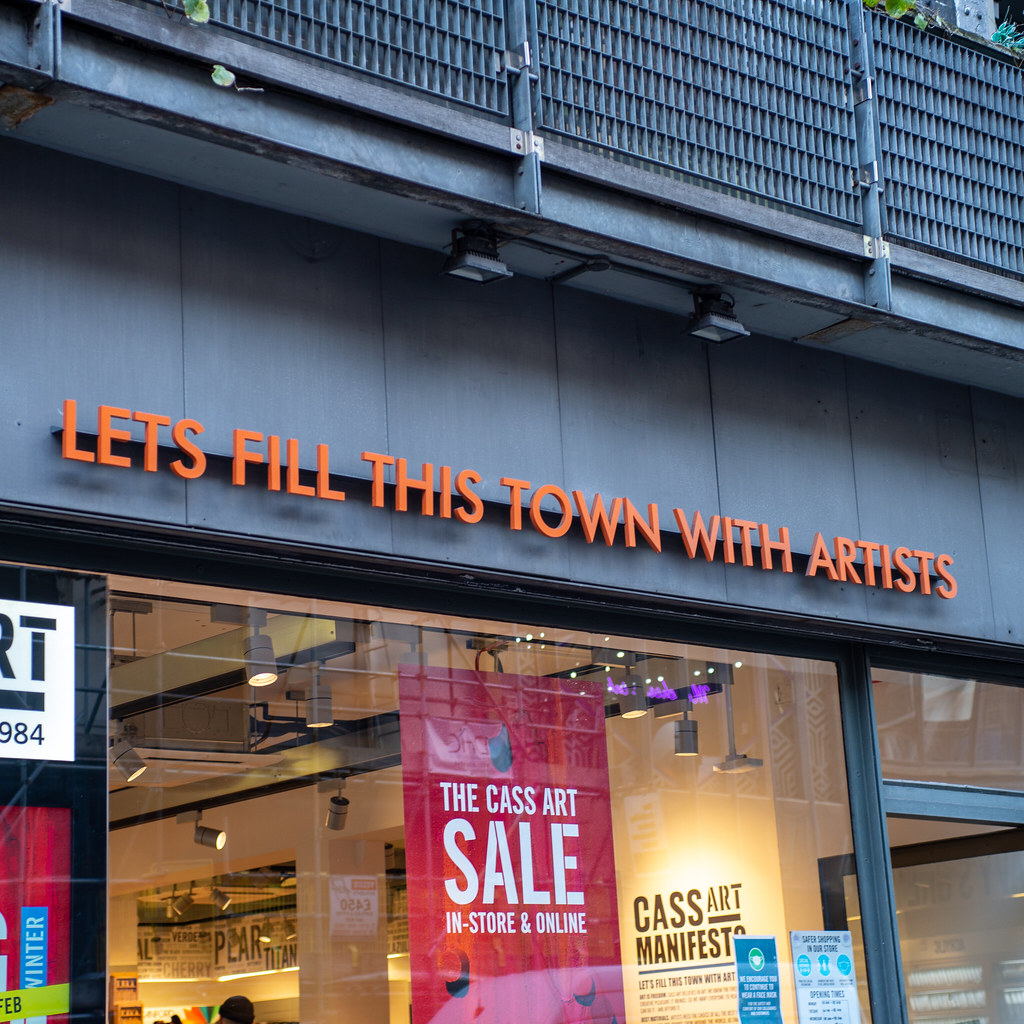The photograph captures the storefront of an art store, characterized by its gray or charcoal-colored exterior. Prominently displayed above the window are the bold, orange words, "Let's Fill This Town With Artists," despite the noticeable absence of an apostrophe in "Let's." Below this inspiring slogan, the window features signage that reads, "The Cass Art Sale, in store and online," and "Cass Art Manifesto," indicating the store's artistic focus. Several smaller stickers are also visible on the window, though their details are too minute to discern. Above the signage, a couple of unlit lights are poised to illuminate the display.